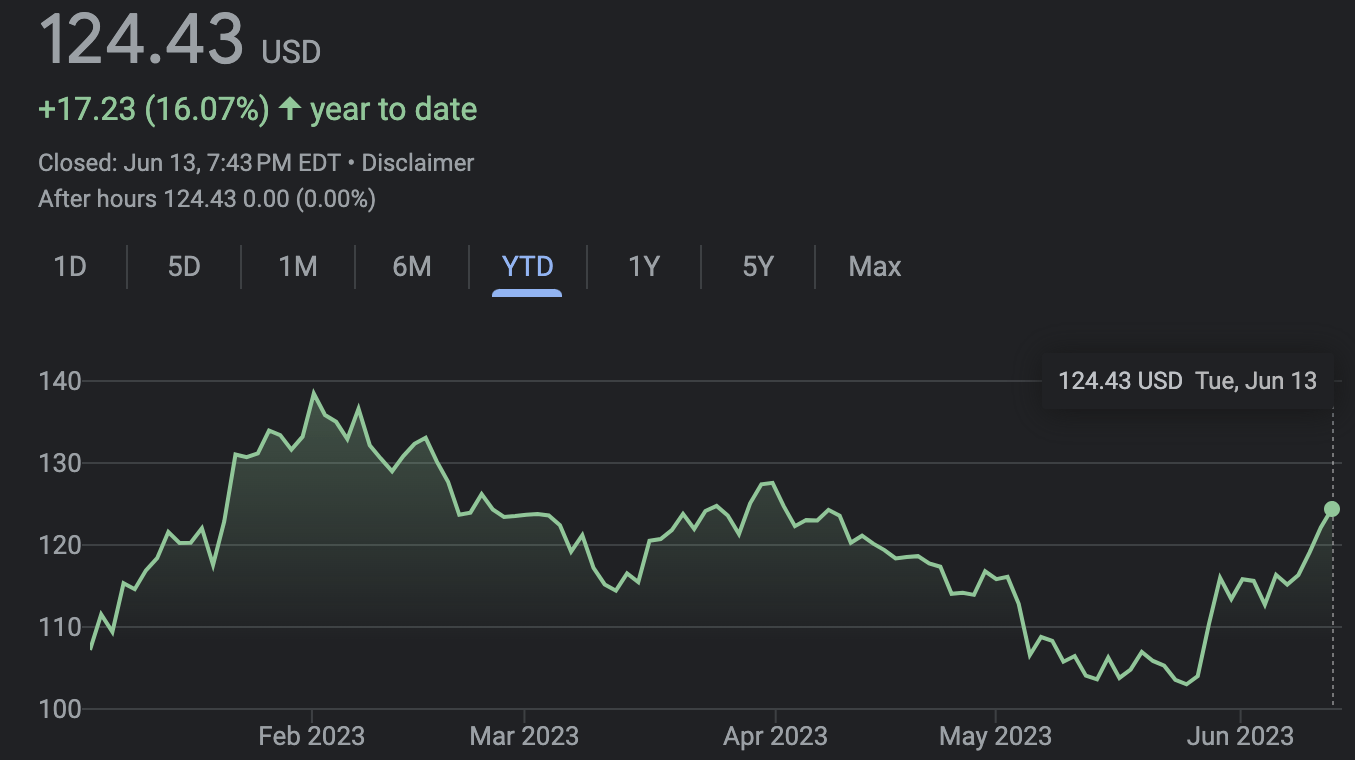The image is a screen capture of a financial chart from an online application or website, showcased within a rectangular window with a black background. The chart's text elements are in a light gray color, with a specific line of text highlighted in pale green for emphasis.

In the upper left corner, the chart displays a value of "124.43 USD," indicating the current stock price or financial measurement. Directly below this, in pale green text, it states "+17.23 (16.07%)" accompanied by an upward arrow, signifying a positive year-to-date performance. Further down, the text "Closed June 3, 7:43 PM EDT • Disclaimer" provides details on the timing and status of the data.

Below the textual information is the chart itself. The vertical axis ranges from 100 to 140, while the horizontal axis marks time from February 2023 through June 2023, with each month clearly labeled. The chart's data points, depicted in green, show a pattern of fluctuations—ascending and descending—corresponding to the financial performance over the specified period.